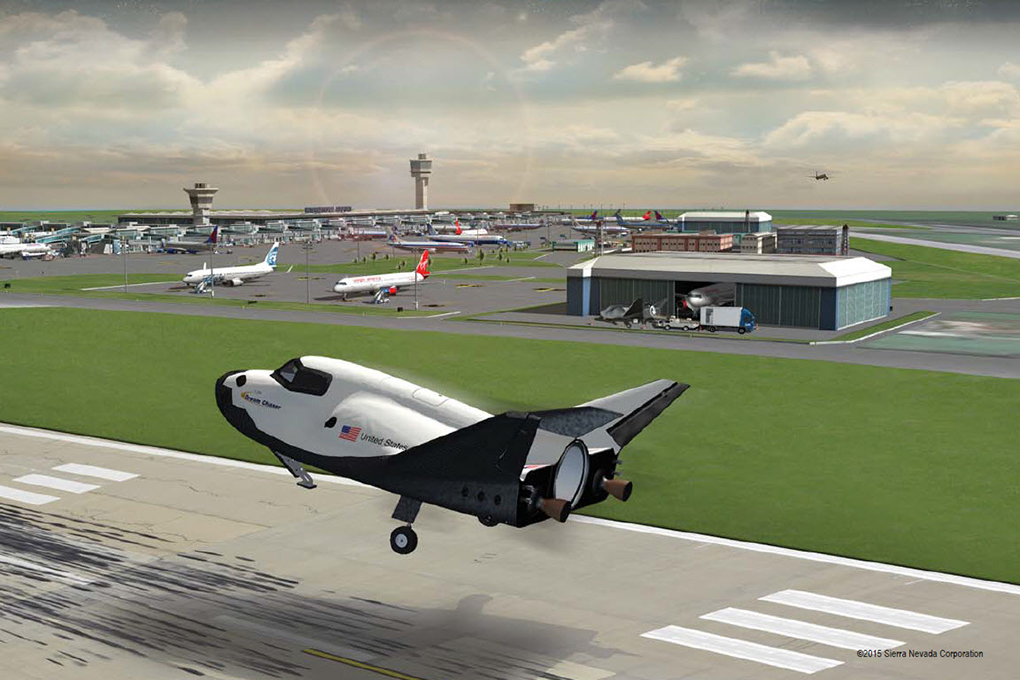The image depicts a highly detailed scene of a hyper-realistic drawing or a screenshot from a video game, showcasing a white and black jet taking off from an airstrip marked by gray pavement with white stripes. The airstrip is bordered by green grass and features a small, garage-like building with a truck nearby. Other planes in various colors, including white, blue, red, and beige, are parked on adjacent airstrips, alongside commercial buildings and a busy parking lot. The airport is equipped with two light gray towers visible in the background. The jet, marked with a small American flag and labeled "United States Dream Chaser," stands as the focal point with its landing gear extended, taking off under a blue-gray sky tinged with brown hues and dotted with fluffy clouds. The bottom right of the image carries a copyright note from Sierra Nevada Corporation, dated 2016.